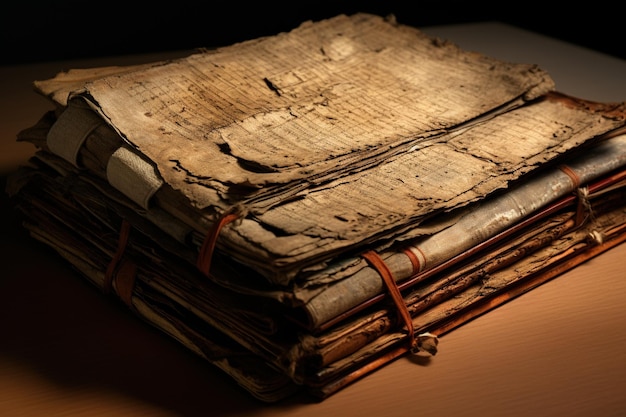The image showcases a collection of very old, ancient documents, possibly including a book at the bottom, stacked in a visually detailed arrangement. The documents exhibit numerous signs of aging, with the top papers appearing especially worn, tattered, and creased, featuring torn and frayed edges indicative of extreme age. The papers and book display a spectrum of earthy tones, ranging from tan to varying shades of brown, with hints of dark orange or rust. Red bands or strings wrap around parts of the stack, although they do not cover the top papers, and some of these strings have a golden bell attached at the ends. The binding elements, including leather straps and white closures, are also evident, especially on the book, enhancing its aged and well-preserved appearance. The entire collection rests on a light brown table, and while some printed text is visible on the documents, it is exceptionally faded and unreadable, adding to the historical and mysterious aura of the scene.